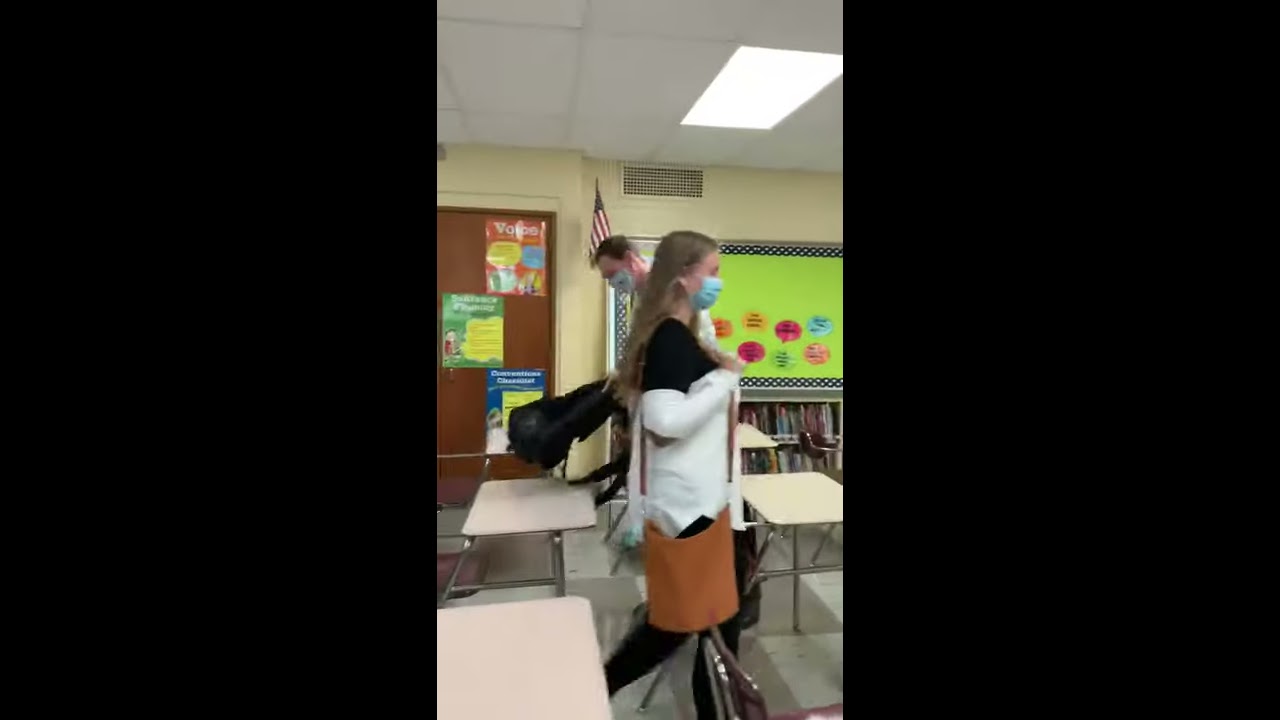This image depicts a slightly blurry scene in a classroom where two adults are present. The shot, framed within a horizontal rectangular picture with wide black bars on either side, centers on a narrow vertical section showing the subjects. Both individuals are wearing blue paper masks, suggestive of the COVID-19 pandemic era.

In the foreground, a woman with long blonde hair is seen walking towards the right. She dons a black and white top, black leggings, and carries a brown purse over her shoulder. Behind her, a man with short brown hair is leaning down, interacting with a black backpack. Both individuals are navigating between several student desks with white tops.

The classroom setting is further detailed by a beige-colored wall in the background, a green-bordered bulletin board adorned with colorful designs, and an American flag extending from the end of a chalkboard. A brown door at the back is decorated with various posters. The ceiling features standard white tiles and a lit rectangular fluorescent light. The floor below them is in a black and white checkerboard pattern, completing the typical classroom ambiance.